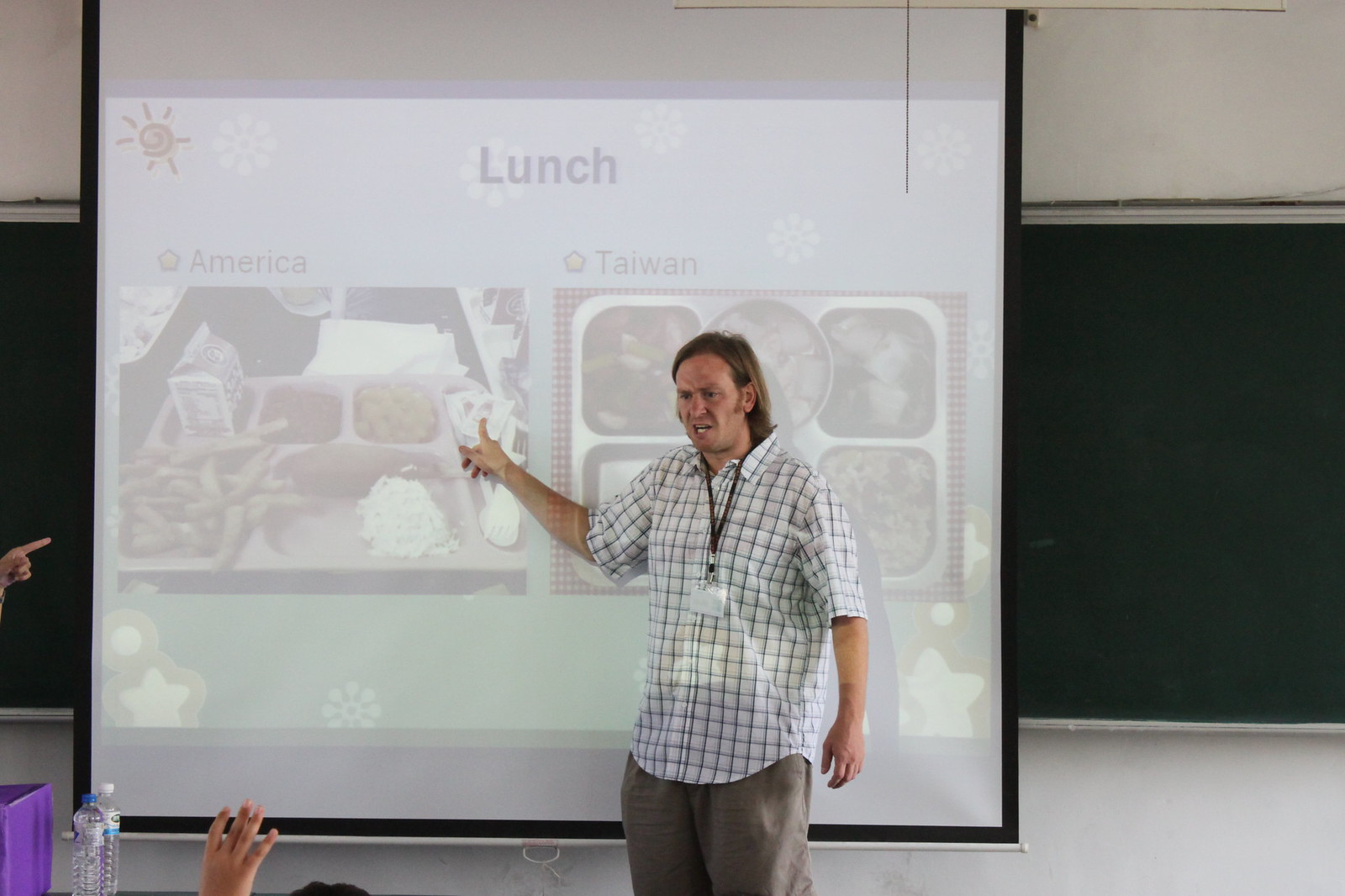A visually engaging classroom scene showcases a professor deeply engrossed in delivering his lecture. The room features pristine white walls, dark-colored doors, and light, possibly white flooring that provide a clean and well-organized ambiance. At the center of the image stands the professor, who is mid-gesture, pointing towards a sizeable projection screen. Dressed in a neatly tucked white checked shirt adorned with brown stripes, a lanyard around his neck, and light brown pants, he maintains a professional yet approachable appearance.

The projection screen, although slightly blurred, clearly displays a title that reads "Lunch," alongside two categories labeled "America" on the left and "Taiwan" on the right. The screen is filled with various images of lunch foods from both regions, hinting at a comparative cultural lesson. Several students, eager to engage, have raised their hands, indicating the interactive nature of the lecture. Despite the slight blur, the image angle suggests an immersive learning environment where students are being educated on the culinary distinctions between American and Taiwanese lunches.